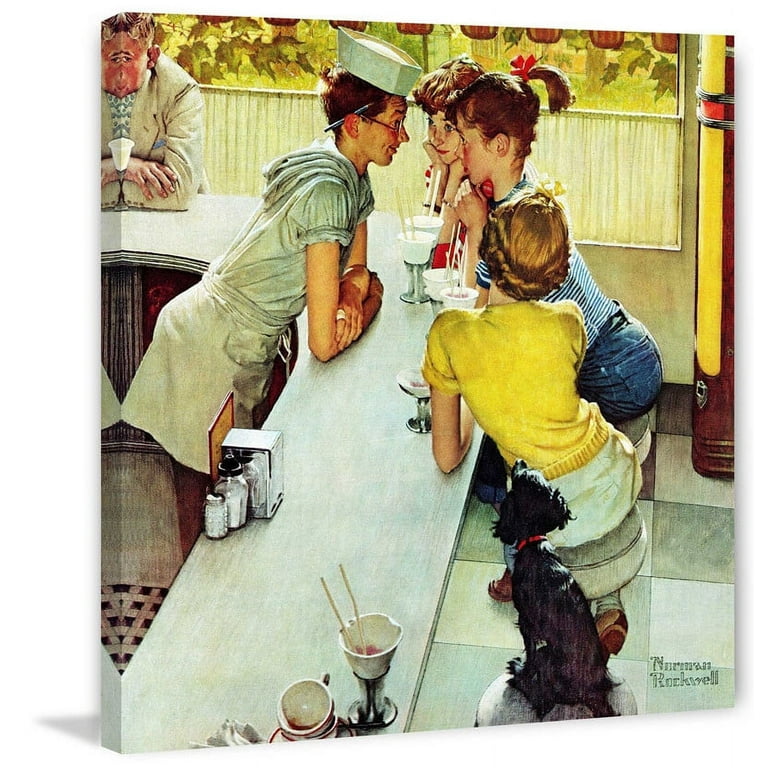This illustration, painted by Norman Rockwell, is a classic scene set in a diner, depicted on a slightly tilted canvas against a solid white background. The composition captures a nostalgic atmosphere with intricate details. A young man, presumably the server, is positioned on the left side of the counter. He is identifiable by his geometrical hat with a rounded top, a white apron, and a pencil tucked behind his ear. His posture is engaged as he leans over the counter, arms resting on it, bending closer to interact with a young girl seated opposite him.

The girl, characterized by her high pigtail and brown hair, dons a blue and white striped shirt. She is accompanied by two other female companions, distinguishable by their unique attire—a red-blue striped shirt and a yellow sweater. They are all absorbed in the moment, their drinks with straws in front of them suggesting they are deep in conversation with the server. Adding to the idyllic charm is a black dog seated near the bottom right corner, gazing up attentively at the girls.

The diner scene is further enriched by a large window in the background, through which some leaves can be glimpsed, hinting at the world outside. There is also another patron partially visible on the left edge of the canvas, adding depth to the social setting. This quintessential Rockwell painting is signed at the bottom right, affirming the artist’s distinctive and heartwarming style.